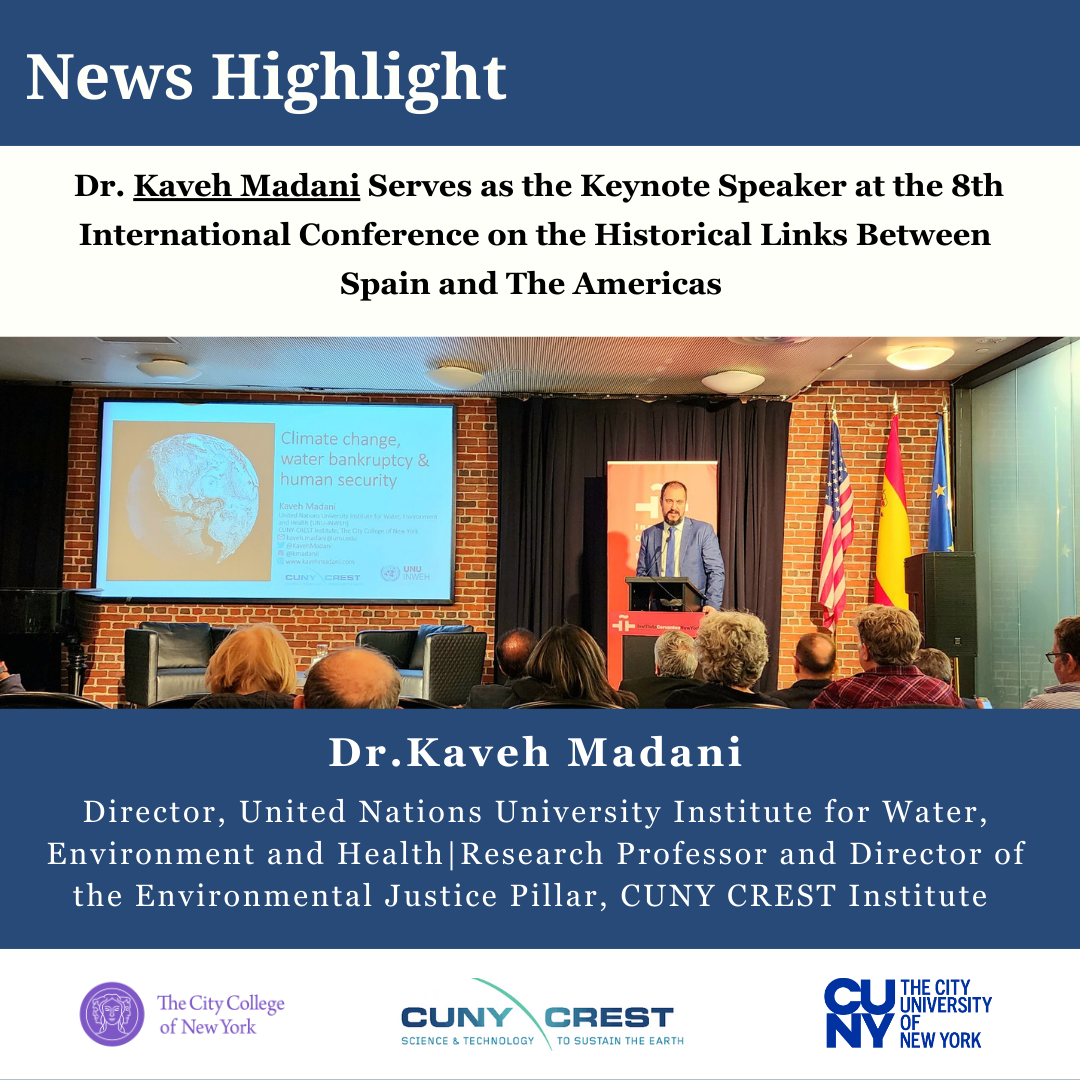The image features a news highlight announcement with a prominent blue banner at the top displaying the words "News Highlight" in white text. Directly below, a white banner with black text states, "Dr. Kaveh Madani serves as the keynote speaker at the 8th International Conference on the Historical Links Between Spain and the Americas." The central photograph captures Dr. Kaveh Madani, attired in a blue suit and tie, delivering a speech at a podium. He is positioned in front of a screen projecting the topics "Climate Change, Water, Bankruptcy, and Human Security." Behind him are the American flag, the Spanish flag, and another unidentified blue flag. The audience, consisting of fewer than a dozen individuals, listens attentively. Below the photo, text in a blue box highlights Dr. Madani's credentials: "Dr. Kaveh Madani, Director, United Nations University Institute for Water, Environment, and Health; Research Professor and Director of the Environmental Justice Pillar at the CUNY Crest Institute, The City College of New York, CUNY."